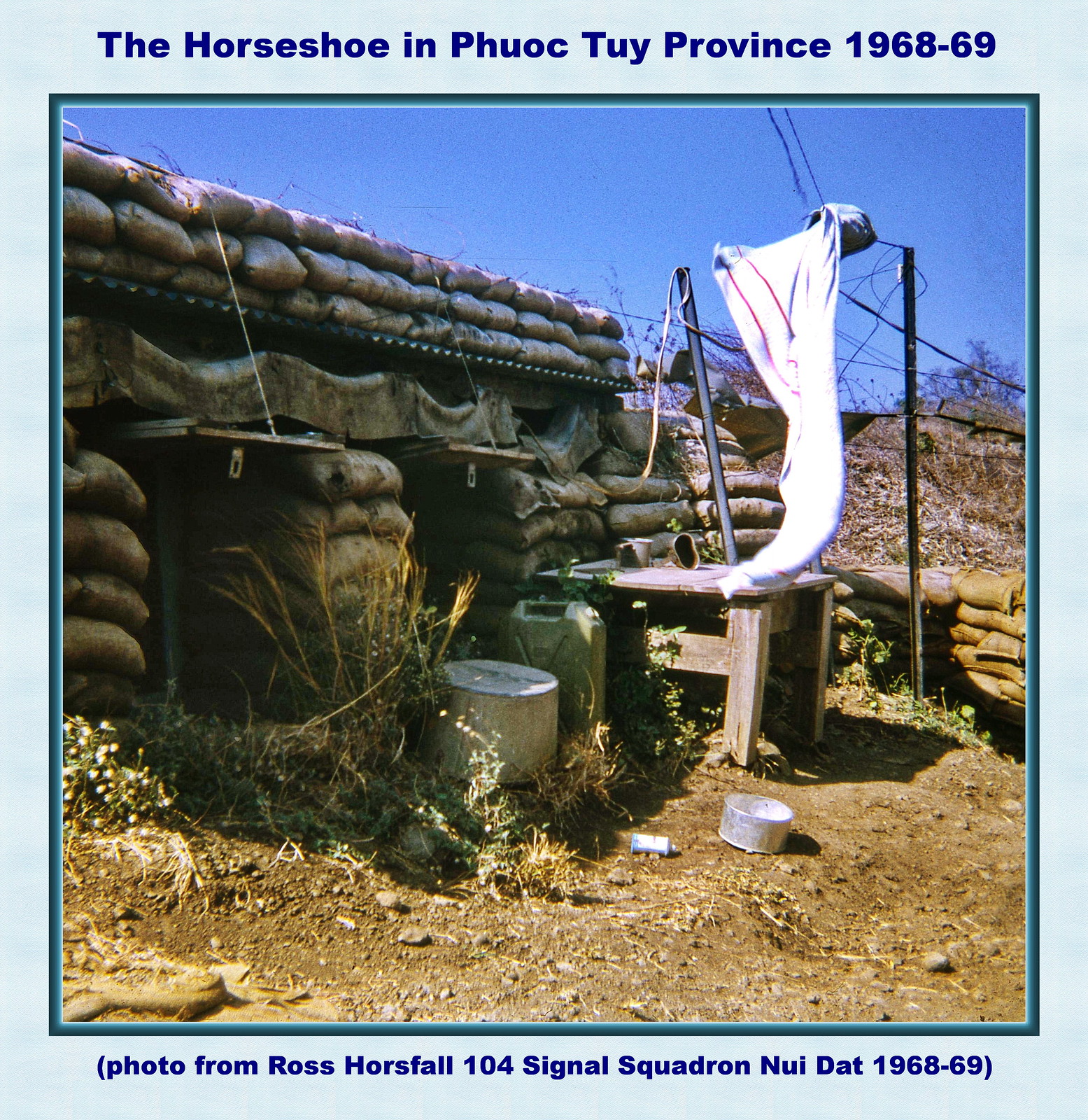The image features a run-down military bunker from the Vietnam War era, specifically located in Phuoc Tuy province, as indicated by the caption that reads "The Horseshoe in Phuoc Tuy province, 1968 to 1969. Photo from Ross Horsfall, 104 Signal Squadron, Nui Dat, 1968 to 1969." The structure is constructed with sandbags piled high to form walls, reinforced by wooden planks that frame the dark interior, giving it the appearance of a house made of sandbags. The roof is a metal sheet covered with more sandbags for added protection.

Outside the bunker, the dirt-covered ground is strewn with various items: a small wooden table, several empty pails, an old gasoline canister, and some metal canisters. A wire strung on poles serves as a makeshift clothesline, with clothing or sheets hanging to dry. Electrical lines and possibly barbed wire are also visible in the vicinity. The area surrounding the bunker appears desolate and dry, with patches of dried grass adding to the overall sense of abandonment.